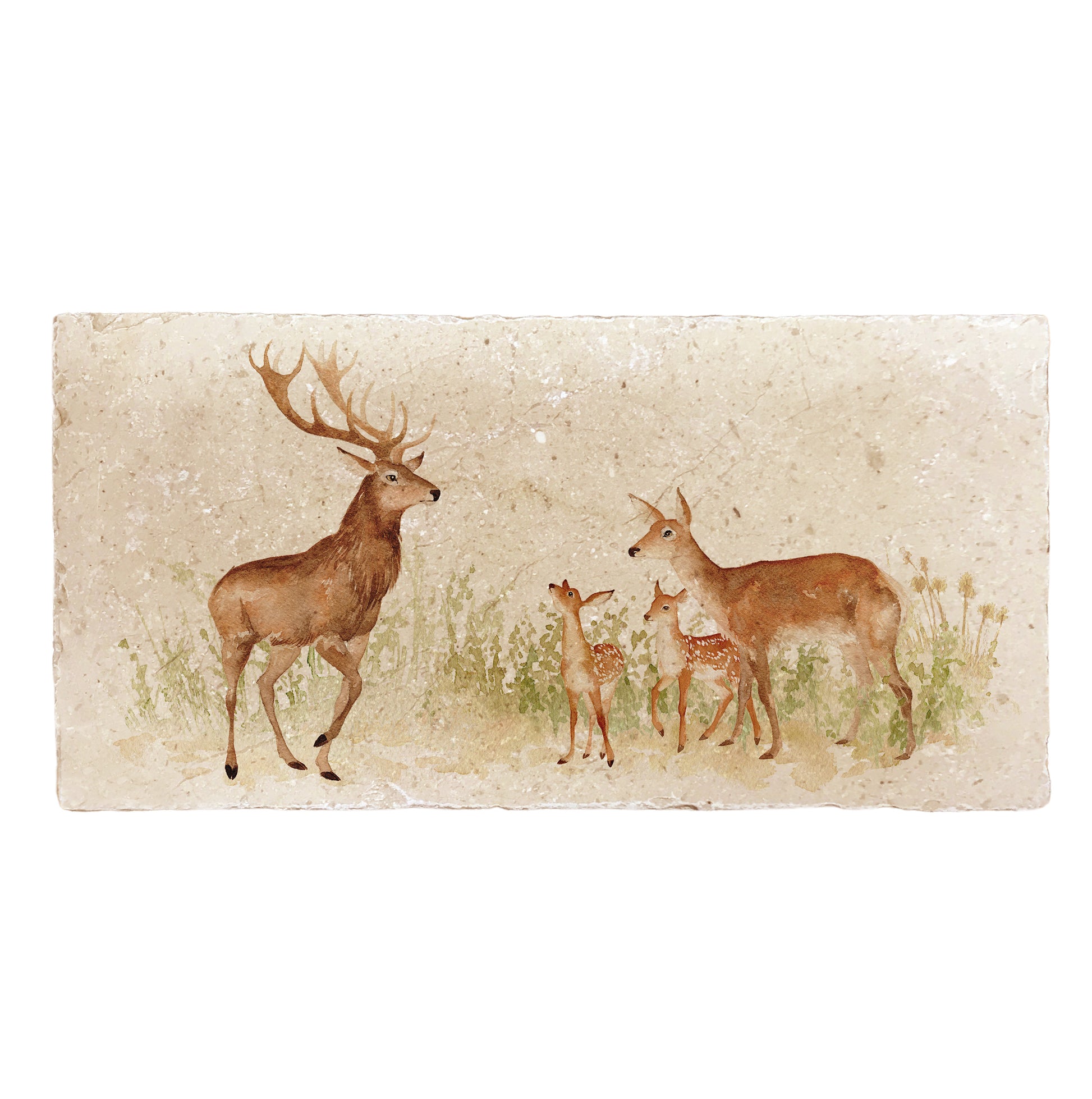This image is a detailed watercolor painting depicting a serene family of deer in a natural setting. The painting, which covers the entire canvas, portrays a large male deer with imposing antlers dominating the left half of the scene, standing gracefully with one foot raised. To the right of the majestic buck are two younger deer and their mother. The younger deer and the doe, all brown with white chests and noticeably smaller and lighter than the buck, gaze towards him. The subtle background is a tan wash with varied splotches and textures, reminiscent of aged stone. The lower half of the painting features delicate brushstrokes and dotting in shades of green and tan, representing tall grass and shrubs that hint at a lush environment. The piece appears meticulously hand-painted on paper or canvas, capturing the tranquil essence of deer in their habitat.